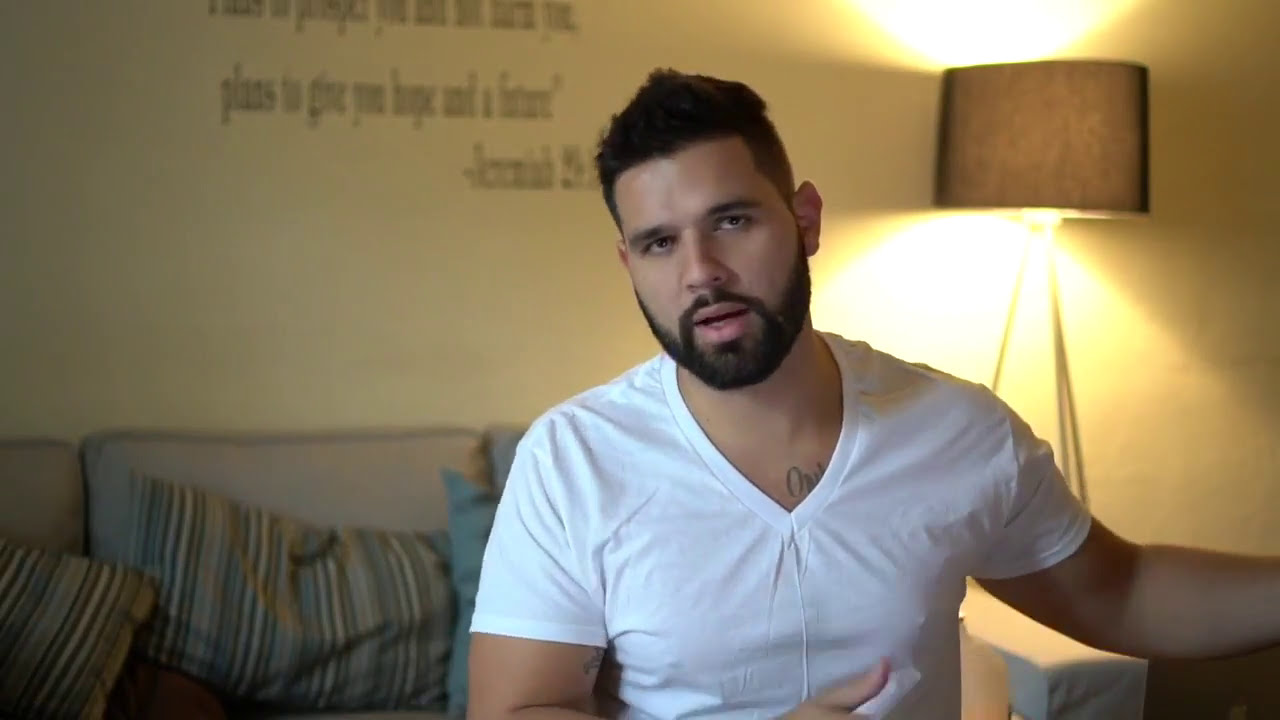This horizontal rectangular photograph captures a light-skinned man sitting in a room, seemingly engaged in conversation, perhaps for a podcast or YouTube video. He has short brown hair, shaved close on the sides and slightly spiked in the center, complemented by a well-groomed brown beard and mustache. He is wearing a white v-neck t-shirt, partially revealing a tattoo on his chest with the letters "O" and "N" visible. A microphone is clipped to his shirt, suggesting he is speaking as his mouth is open. His right arm is bent in front of him while his left arm extends out of frame. Behind him, a beige couch with striped pillows—decorated with vertical stripes in green, brown, and beige—sits against a light brown wall. On the right side of the image, a lit lamp with a brown shade casts a warm yellow light, illuminating a quote on the wall. The quote is partially legible, ending with "plans to give you hope and a future" followed by a reference to Jeremiah.